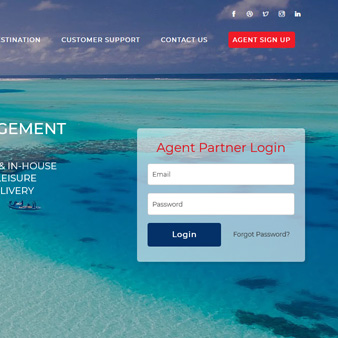The image displays the upper quarter of a webpage's homepage, featuring a tropical, serene setting with light, clear blue waters. The background showcases shallow waters with visible land formations near the seafloor and a small boat with people onboard. Prominently displayed in the foreground is the "Agent Partner Login" section, which includes fields for email and password, a large blue login button, and a "Forgot Password" option. The navigation links at the top of the page include "Destination," "Customer Support," "Contact Us," and "Agent Sign Up." In the top-right corner, social media icons for Facebook, Twitter, LinkedIn, Instagram, and an indiscernible platform are also visible.